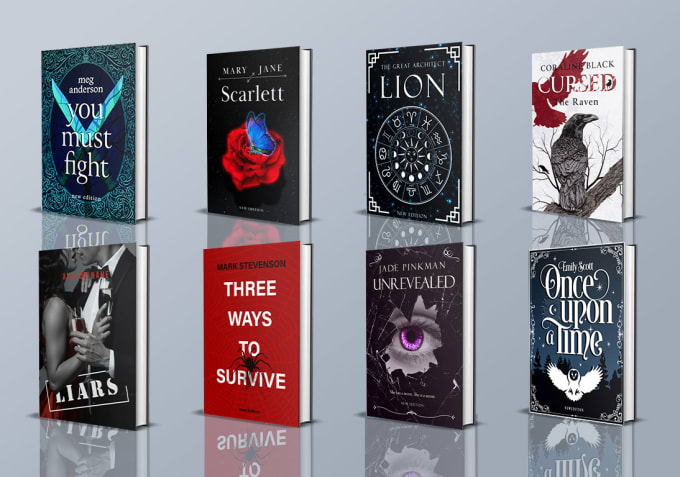In this image, there are eight books organized in two rows of four, placed on a reflective gray surface that casts clear reflections below each book. The books are as follows:

1. "You Must Fight" by Meg Anderson, featuring a blue wing-like shape and a green-blue design on the cover.
2. "Scarlet" by Mary Jane, adorned with a red rose on a black background.
3. "The Great Architect Lion," which has a black background and a circular object displayed prominently.
4. "Cursed, The Raven" by Coraline Black, showcasing a picture of a raven perched on a tree branch, against a white cover.
5. "Liars," depicting a couple about to kiss.
6. "Three Ways to Survive" by Mark Stevenson, featuring a red cover with a spider motif.
7. "Unrevealed" by Jade Pinkman, with a black cover and a see-through cut-out revealing a pink eye.
8. "Once Upon a Time" by Emily Scott, illustrated with a white owl against a blue background with darker shades at the bottom.